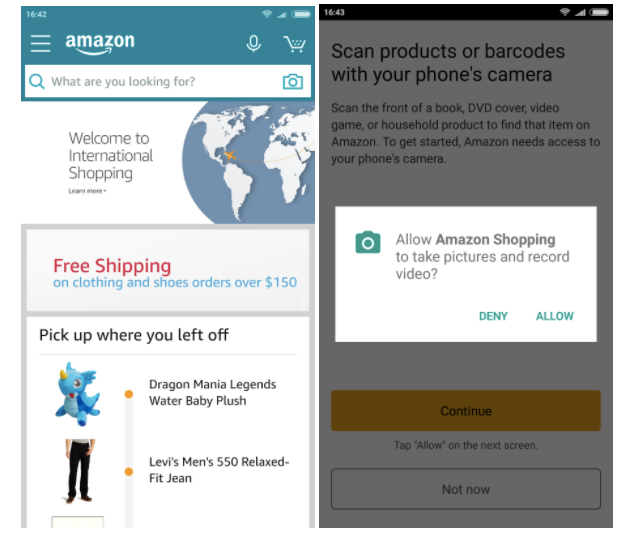The image features two distinct screenshots from the Amazon Shopping app. 

On the left side, the Amazon home page is displayed upon opening the app. The interface welcomes users to international shopping, with a highlighted offer of free shipping on clothing and shoe orders over $150. Below this, the page prompts users to "Pick up where you left off" and showcases various products including a "Legends Baby Plush" toy and a pair of "Levi's Men's 550 Relaxed Jeans."

On the right side, the screenshot captures a pop-up message requesting camera permissions. The prompt reads, "Allow Amazon to take pictures and record video" with options to either "Deny" or "Allow" the app access to the camera for scanning products or barcodes. The slightly blurred background reveals the Amazon interface, indicating that the permissions request is integrated into the shopping experience. Users have additional options to "Continue" or select "Not now," allowing them to enable this security setting on their phone if they wish to use the camera to look up products.